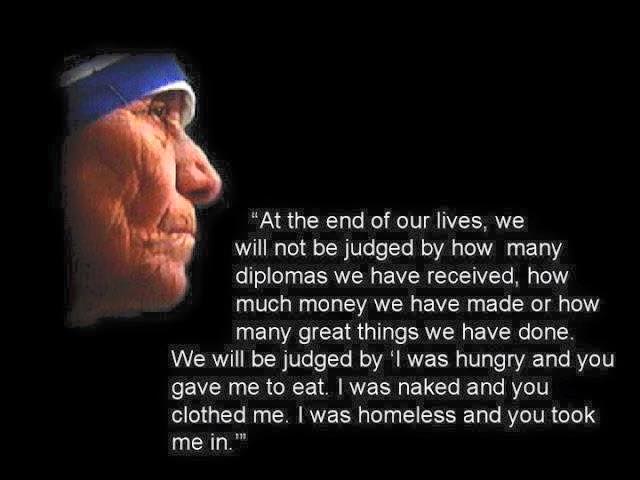The image features a black background with a side profile of Mother Teresa's face on the upper left-hand side, showing the right side of her face. She is depicted wearing her traditional religious habit. The right-hand side of the image contains a quote attributed to Mother Teresa in small white font: "At the end of our lives, we will not be judged by how many diplomas we have received, how much money we have made, or how many great things we have done. We will be judged by, I was hungry, and you gave me to eat. I was naked, and you clothed me. I was homeless, and you took me in." The overall design is simple and solemn, with no additional elements apart from the photograph and the text.